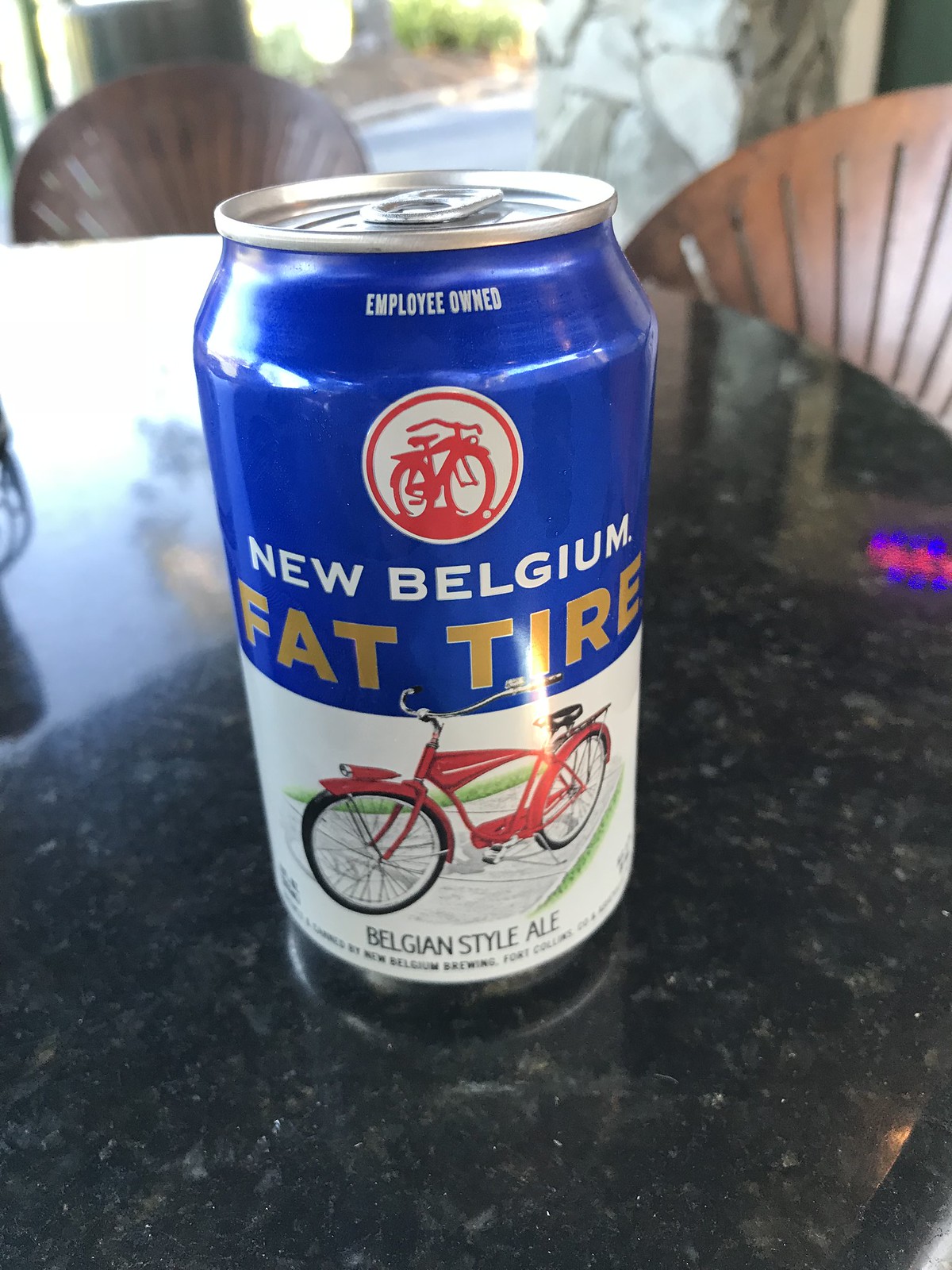This digital photograph prominently features an unopened aluminum can of New Belgium Fat Tire beer, showcasing a striking design with blue and white stripes. The can's top half is blue, transitioning to white at the bottom, with the top remaining silver and uncracked. In white lettering at the top, it reads "Employee Owned." A central focal point is the large white bezel with a red bicycle and a red line inside the circle. Beneath this icon, the words "New Belgium" are inscribed in white, followed by "Fat Tire" in bold yellow letters. Below this, against the white background, is another retro-styled red bicycle with black wheels. Further text beneath the second bicycle states "Belgian Style Ale" in black letters. 

The can is positioned in the center of a black granite countertop with specks of white, gray, and brown. The background includes two brown chairs with slits resembling a fan back, hinting at a sunny outdoor setting. Greenery visible through what appears to be a window and a white and gray marble wall add depth to the scene. There’s also an element that looks like a table with a white tablecloth, along with faint imagery of a wicker or wooden chair, contributing to the overall ambiance.